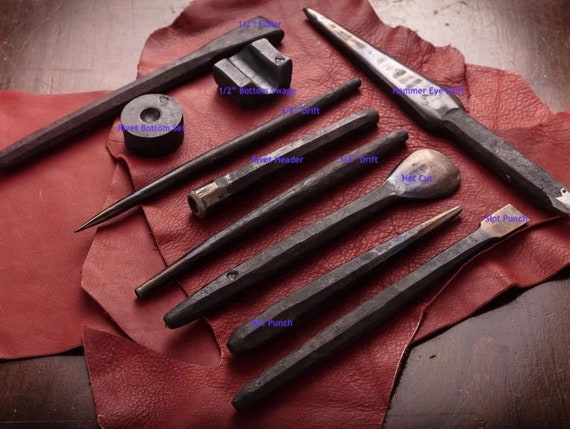This detailed photograph captures a close-up of ten various leatherworking tools neatly arranged on a piece of red leather, which itself rests atop a dark brown wooden countertop. The tools, made from heavy metal and exhibiting signs of wear and rust, suggest extensive use and age. Each tool is labeled with small purple text, though the labeling can be somewhat difficult to decipher. Clearly visible labels include "half inch bottom swap," "hot cut," "slot punch," and "hammer eye." The assortment features different types of awls, punches, and other specialized tools, such as a spoon-shaped tool and a knife-like implement. This image appears to serve as a descriptive guide, showcasing the specific names and appearances of each tool used in leatherworking.